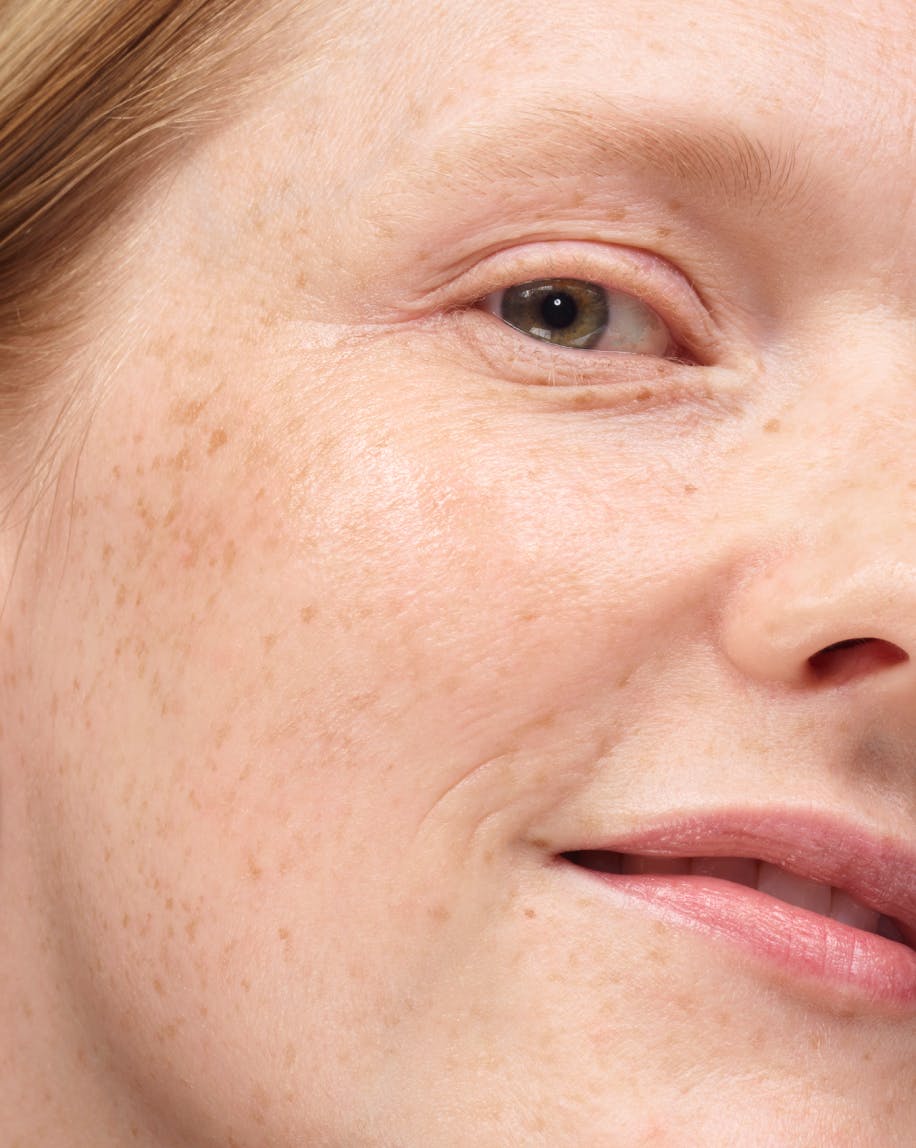This photograph showcases a close-up of a woman's face, heavily zoomed in on the right side. The woman has a light skin tone adorned with numerous brown freckles, which are prominently visible on her face and upper neck. She has a partial smile that reveals the top row of her white teeth and her lips are a soft pink hue. Her head is tilted slightly to her left, the right side of the image, while her striking green eyes gaze directly forward. Her thin eyebrows are a reddish-blonde color, complementing her fiery orange hair, of which only a small portion is visible in the shot. The focus on her face is so tight that her forehead and most of her hair's length are out of frame, emphasizing her facial features and freckled complexion.